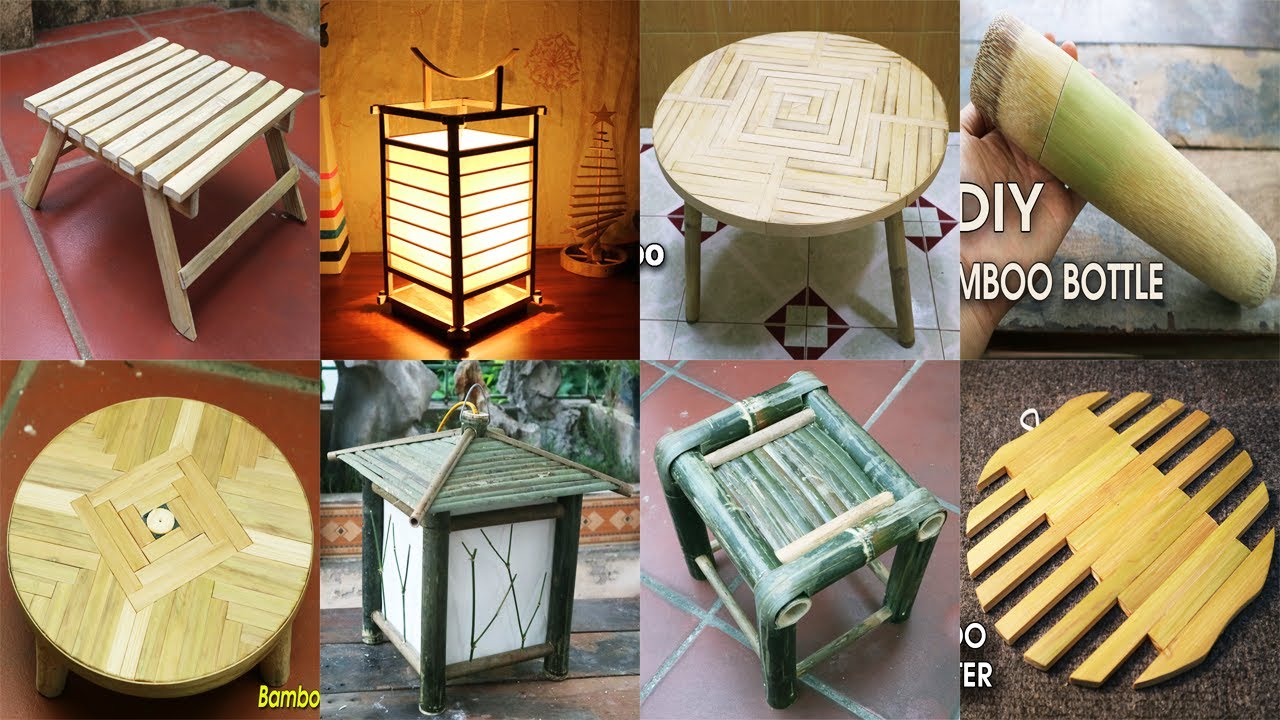This advertisement for DIY bamboo creations features a detailed photo collage of eight individual bamboo items, showcasing the versatility and aesthetic appeal of bamboo in home furniture and accessories. The collage, arranged in two rows of four, highlights the variety and craftsmanship involved in these projects.

On the top row, from left to right, is a square bamboo stool made of slats, followed by a delicate paper lantern with a bamboo frame, then a round bamboo stool with tightly arranged slats forming a square pattern. The last image on the top row is a DIY bamboo bottle, which appears as a tannish-yellow tube with a green stripe near one end.

The bottom row begins with either a round bamboo stool or coffee table, exhibiting intricate engraving on its surface. Next is another paper lantern with a bamboo frame, this one adorned with a roof-like structure and additional delicate details. The following image is a green square stool, accented with tan and black colors. Finally, there is a bamboo trivet, which could also function as a decorative hanging piece due to its attached loop.

The items are presented with varying shades of brown and tan bamboo, creating an eye-catching and cohesive display. The collage effectively illustrates the creative and practical potential of bamboo in DIY projects.